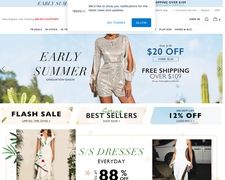The screenshot appears to capture the homepage of an online shopping website focused on women's casual wear, particularly dresses. The image is somewhat blurry, making some text hard to read. At the top, there's a prominent header in black text over a sky-blue background, likely announcing an "Early Summer Sale" or similar event.

A pop-up box dominates the center, promoting an email list subscription with an enticing offer. Though the description is not fully legible, it suggests subscribers may receive benefits. The pop-up features two buttons: a white "No Thanks" and a blue "Join Now."

Centered in the image is a model posed against a desert backdrop with cacti, wearing a stylish, shimmery long-sleeve shirt paired with matching shorts. To her right, there's text highlighting a 20% discount and free shipping on orders over $109.

Beneath the model, there are sections for "Flash Sale," "Bestsellers," and "12% Off." Each section includes clickable buttons to explore the respective deals. Following these, a series of images showcases various fashion styles: one features a woman in a white dress with floral accents, another promotes an 88% discount on "SS Dresses," and a third shows a woman stepping out of a car in a white dress with distinct cuts and slits along its sides.

Overall, the website appears vibrant, focusing on trendy summer fashion with multiple enticing discounts and offers.